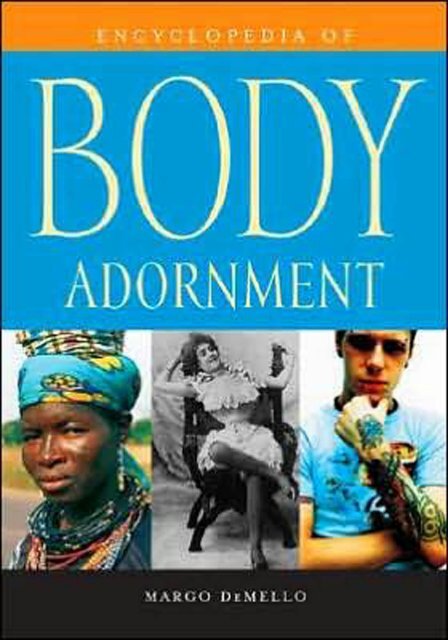The image depicts the cover of a book titled "Encyclopedia of Body Adornment" by Margot de Mello. The cover features a vibrant color scheme with the top portion in orange and the bottom in blue, showcasing the book's title in bold, white letters. Below the title are three distinct images: on the left, an image of an Aboriginal woman adorned with various piercings, wearing a colorful array of beaded necklaces and a cloth wrap with yellow floral patterns on her head; in the center, a black-and-white photograph of a World War I-era woman in a tightly-laced corset and white dress; and on the right, a contemporary man with piercings on his eyebrows and tattoos on his left forearm, wearing a light blue shirt. The author’s name, Margot de Mello, is displayed at the bottom of the cover in white letters against a black background. The image has noticeable compression artifacts, affecting its overall quality.